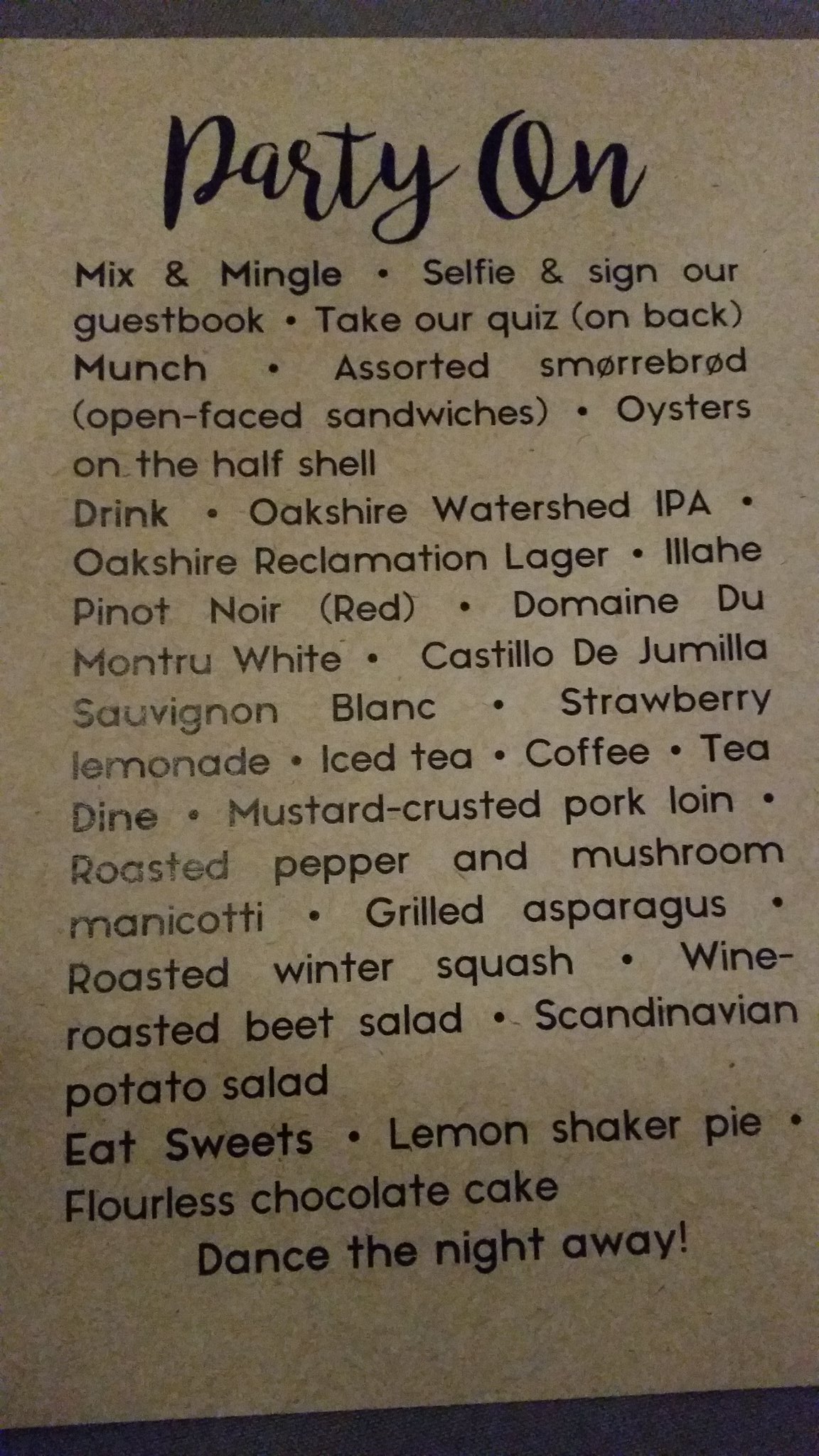In this black-and-white image, we see a detailed sign outlining the various elements of a social event, possibly a cocktail hour, dinner party, or gathering. The top of the sign features the phrase "Party On," which might be the name of the event or venue. Below, it encourages guests to "Mix and Mingle," "Selfie and Sign our Guestbook," and "Make our Quiz." 

The menu is categorized into different sections, starting with appetizers such as "Assorted S'more Board," "Open-Faced Sandwiches," and "Oysters on the Half Shell." For beverages, the offerings include "Oakshire Watershed IPA," "Oakshire Reclamation Lager," "Ila Hay Pinot Noir," "Domaine du Montreux White," "Castilla de Jumilla Sauvignon Blanc," "Strawberry Lemonade," "Iced Tea," "Coffee," and "Tea."

The dinner section, under the title "Dine," lists "Mustard Crusted Porkloin," "Roasted Pepper and Mushroom Manicotti," "Grilled Asparagus," "Roasted Winter Squash," "Wine Roasted Beet Salad," and "Scandinavian Potato Salad."

For desserts, under "Eat Sweets," the menu features "Lemon Shaker Pie" and "Flourless Chocolate Cake." 

The sign concludes with a call to action to "Dance the Night Away," hinting at a fun-filled conclusion to the event. This meticulous menu and schedule outline promise a delightful and well-organized gathering for attendees.